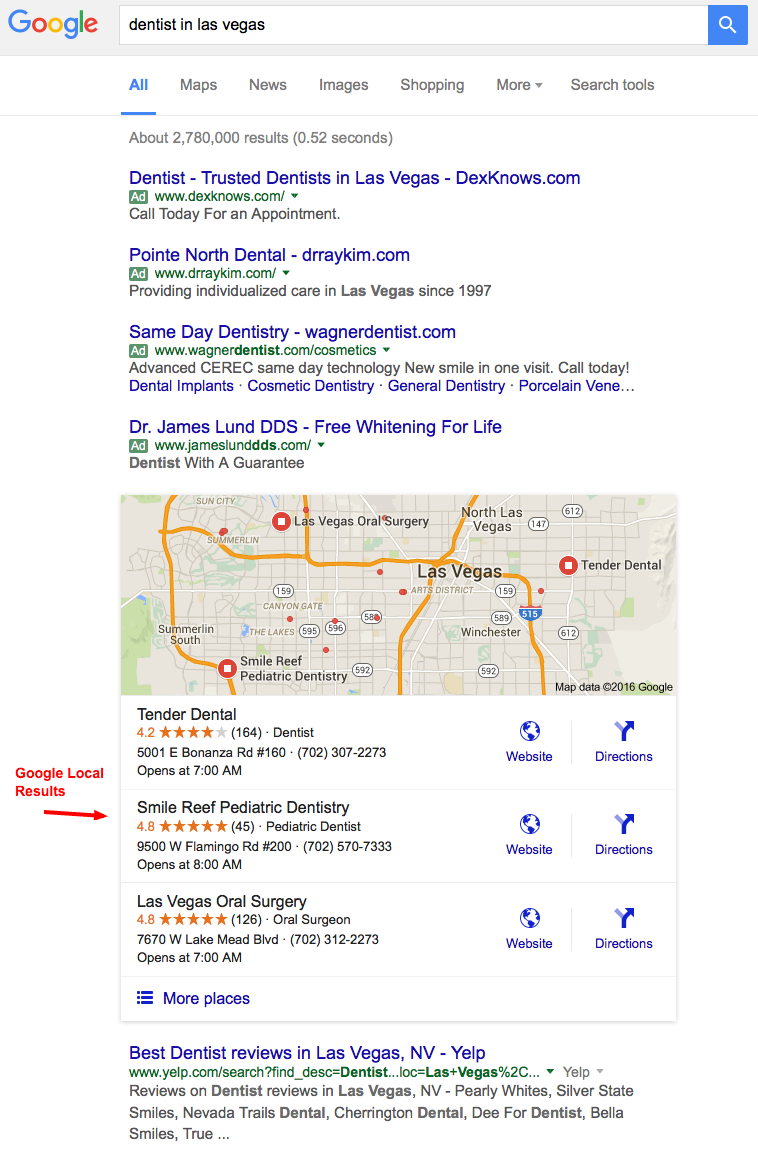The image displays a Google search results page for dentists in Las Vegas, Nevada. At the top, we see the familiar Google logo with the search bar below it, indicating the location as Las Vegas. The search has yielded approximately 2,780,000 results. The options "All," "Maps," "Images," and "More" are visible for further refining the search.

The first result is for Tristan, a dentist in Las Vegas, with accompanying text notes, comments, and advertisements prompting users to call today for an appointment. Next, there is a listing for North to Dental, featuring same-day dentistry services, and Dr. Duong Vuong, who offers teeth-whitening for life. 

A map pinpointing various dental locations in Las Vegas is included, featuring several marked spots. One notable area has a red square with a red circle containing a white square inside it, labeled "Tender Dental." Other identified practices include "Las Vegas Oral Surgery," and "Smile Reef Pediatric Dentistry."

The map also highlights Google Local listings with reviews and ratings: Tender Dental is rated 4.2 stars, Smile Reef Pediatric Dentistry 4.8 stars, and Las Vegas Oral Surgery 4.8 stars. The image effectively captures detailed search results for dentist reviews in Las Vegas, Nevada.